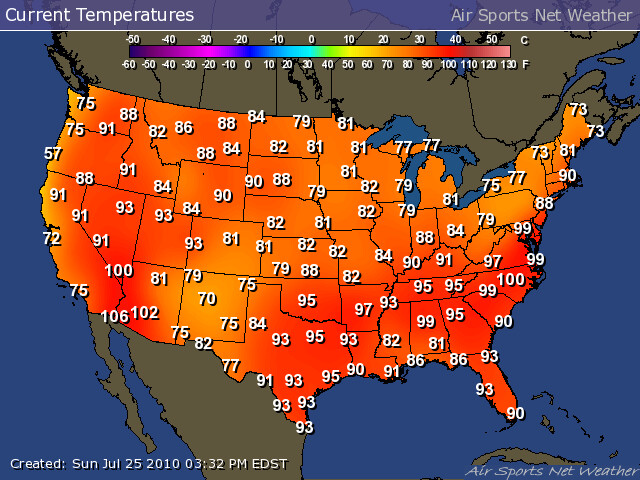The image is a detailed weather map of the United States, reminiscent of those seen on weather channels or their websites. Across the top, a banner reads "Current Temperatures" in bold on the left, and "Airsports Net Weather" on the right in a grayed-out font. The map features a color legend on the side that transitions from dark purple to light pink, representing temperatures from -50°C to 50°C (or -60°F to 130°F). The United States is predominantly colored in shades of orange and red, indicating widespread warmth, with specific areas highlighted in red for higher temperatures. The surrounding ocean is a water blue, while the areas below the U.S., including parts of Mexico, are grayed out. Scattered across the map are white-font numerals denoting specific temperatures in different locations, such as "Houston 95," "LA 75," and "New York 90," though city names are not explicitly labeled. At the bottom left, there is a timestamp that reads "Created Sunday, July 25, 2010, at 3:32 PM EDST," and a subtle "Airsports Net Weather" watermark is present at the bottom of the map.